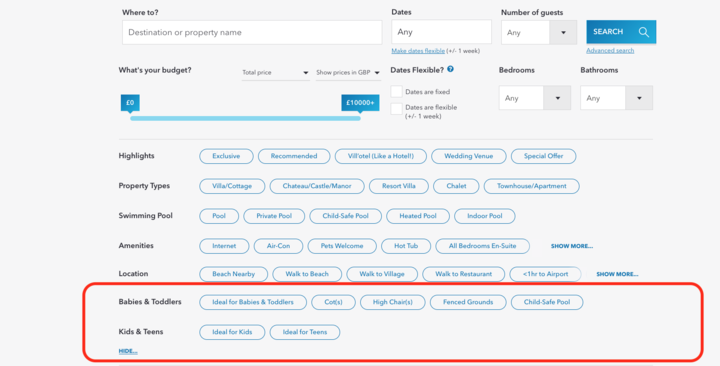The image showcases a detailed search interface with a predominantly gray background. At the top, there's a heading that reads "Where to?" accompanied by a search box labeled "Destination or property name." Below are various search parameters, such as "Dates," "Number of guests," and a "Search" button. There are additional filters for "Budget," "Dates found," "Bedrooms," and "Bathrooms" to refine the search further.

To ensure your search results are accurate, the interface highlights key criteria including "Property types," "Swimming pool availability," "Amenities," and "Location." 

A distinct red box is prominently featured, containing sections tailored for family-friendly travel. It lists categories like "Babies and toddlers" and "Kids and teens." Under "Babies and toddlers," it notes properties with a "Fenced ground" and a "Child-safe pool," along with options for a "High chair" and a "Cot." The next section focuses on "Kids and teens," indicating properties ideal for these age groups. 

This interface seems designed to cater to various family needs, ensuring a comprehensive and tailored search experience.